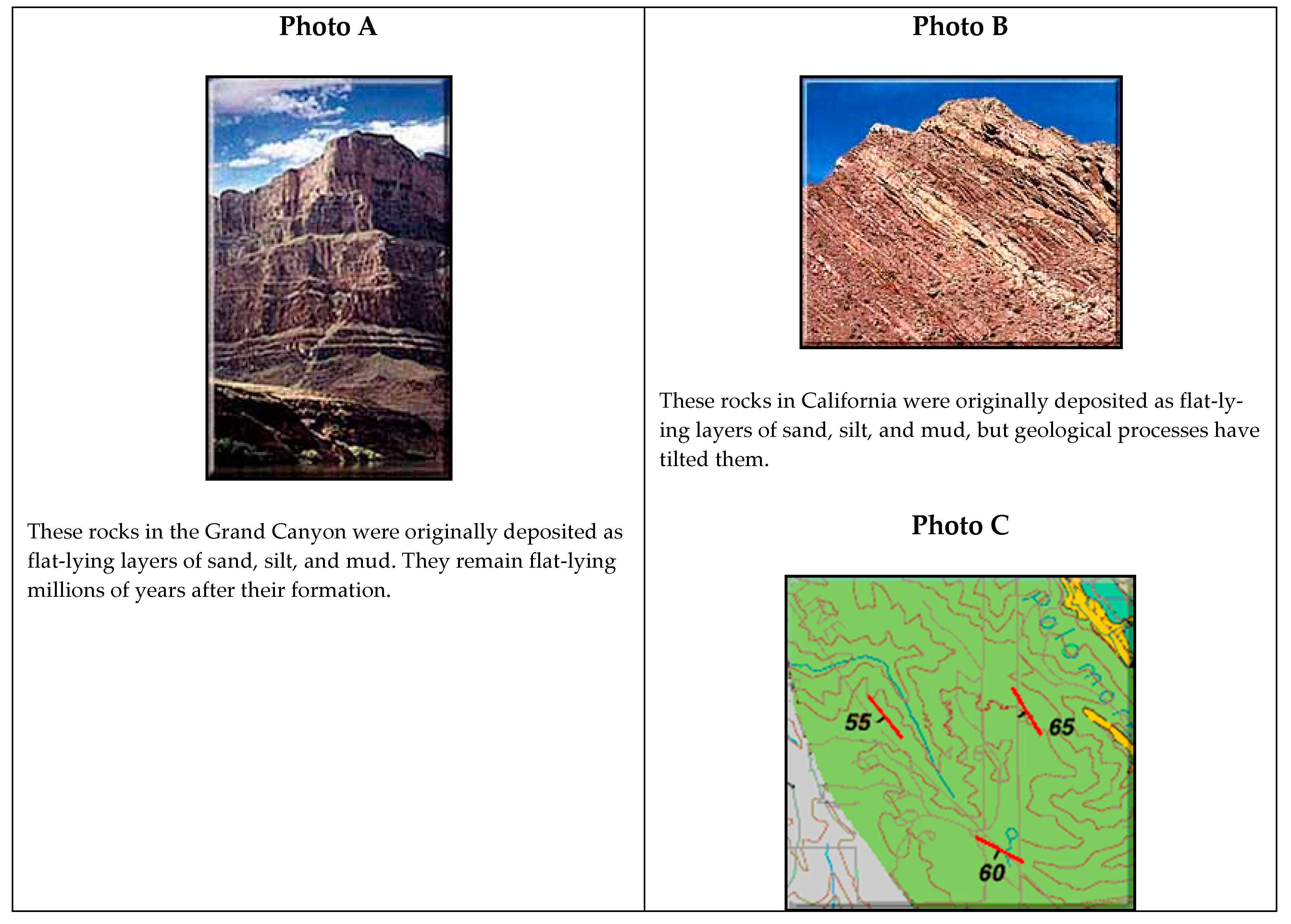The image is an educational collage likely intended for an online resource or digital textbook, featuring a series of photographs and a digitally rendered map, each accompanied by descriptive text. The entire layout includes a thin black border around the edge and a vertical dividing line down the center.

On the left half, labeled as Photo A, there's a large rectangular photograph depicting the strata of the Grand Canyon. This daytime image captures the steep cliffs and visible rock layers extending up to a sky dotted with clouds. The caption underneath explains that these rock layers were originally deposited as flat layers of sand, silt, and mud, and have remained flat-lying for millions of years.

On the right half, the layout is divided into two smaller sections. The upper section, labeled Photo B, presents another geological formation in California. This photograph, also taken during the day, features striated rock layers that have visibly tilted due to geological processes. The brown hues of the tilted layers contrast against a blue sky with fewer clouds than in Photo A. The caption reiterates the rock's originally flat-lying deposition and the subsequent tilting caused by geological forces.

Below Photo B, the lower section is labeled Photo C and contains a digitally produced map. Predominantly green, this map illustrates topographic details, possibly indicating elevations or geographical features with contours and red lines. The numbers 55, 65, and 60 are marked, likely denoting degrees of angle or some metric related to the mapped region's features.

This detailed layout serves as an illustrative resource showcasing both real-life geological formations and abstract geographical data.